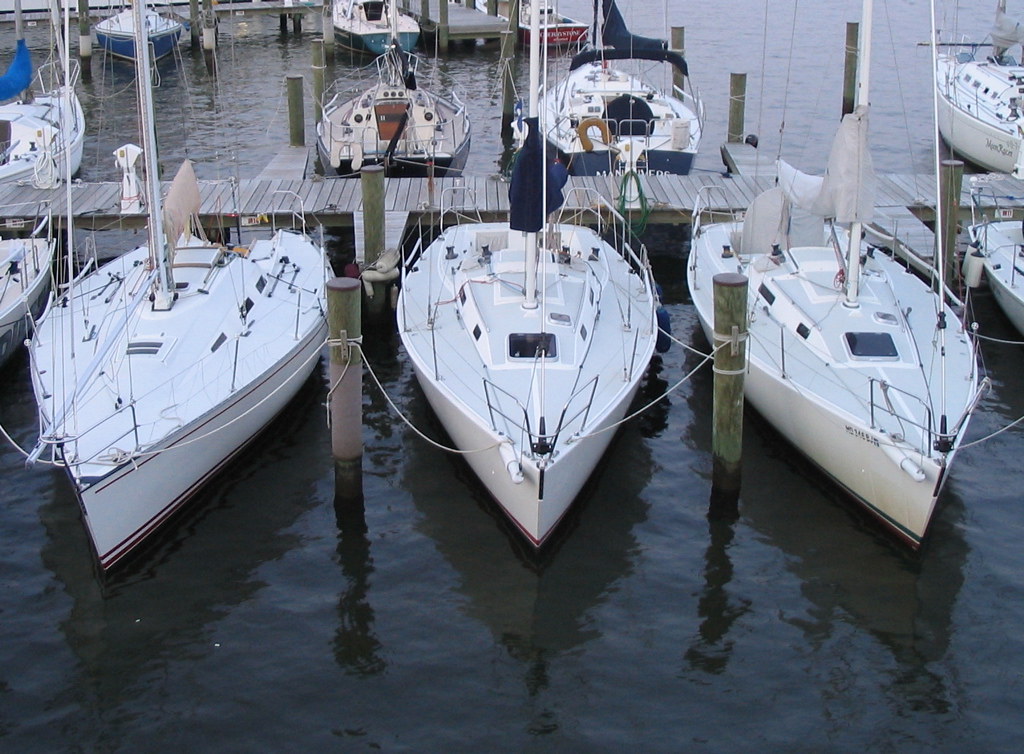This detailed image captures a marina with multiple boats docked along a faded wooden pier. The water, dark and almost black with a few ripples, reflects the light subtly. In the foreground, three white sailboats are prominently featured, each tethered to green-discolored wooden beams. The sails are down, with the boat on the left displaying a tan sail, the one in the center a blue sail, and the one on the right a white sail. The rightmost boat may have some text on its left side, though it's illegible.

Beyond these, parts of two additional boats are visible flanking the main trio, hinting at an array of docked vessels. Moreover, in the upper portion of the image, several more boats are seen, though less prominently. These boats, some facing away from the viewer, have their sails down: notable ones include a blue and white boat, an aqua blue and white boat, a black and white boat, a dark blue and white boat with some white lettering, and a white boat on the far right. Another dock appears in the background, with a distinctive red boat parked nearby, adding a splash of color to the serene scene.